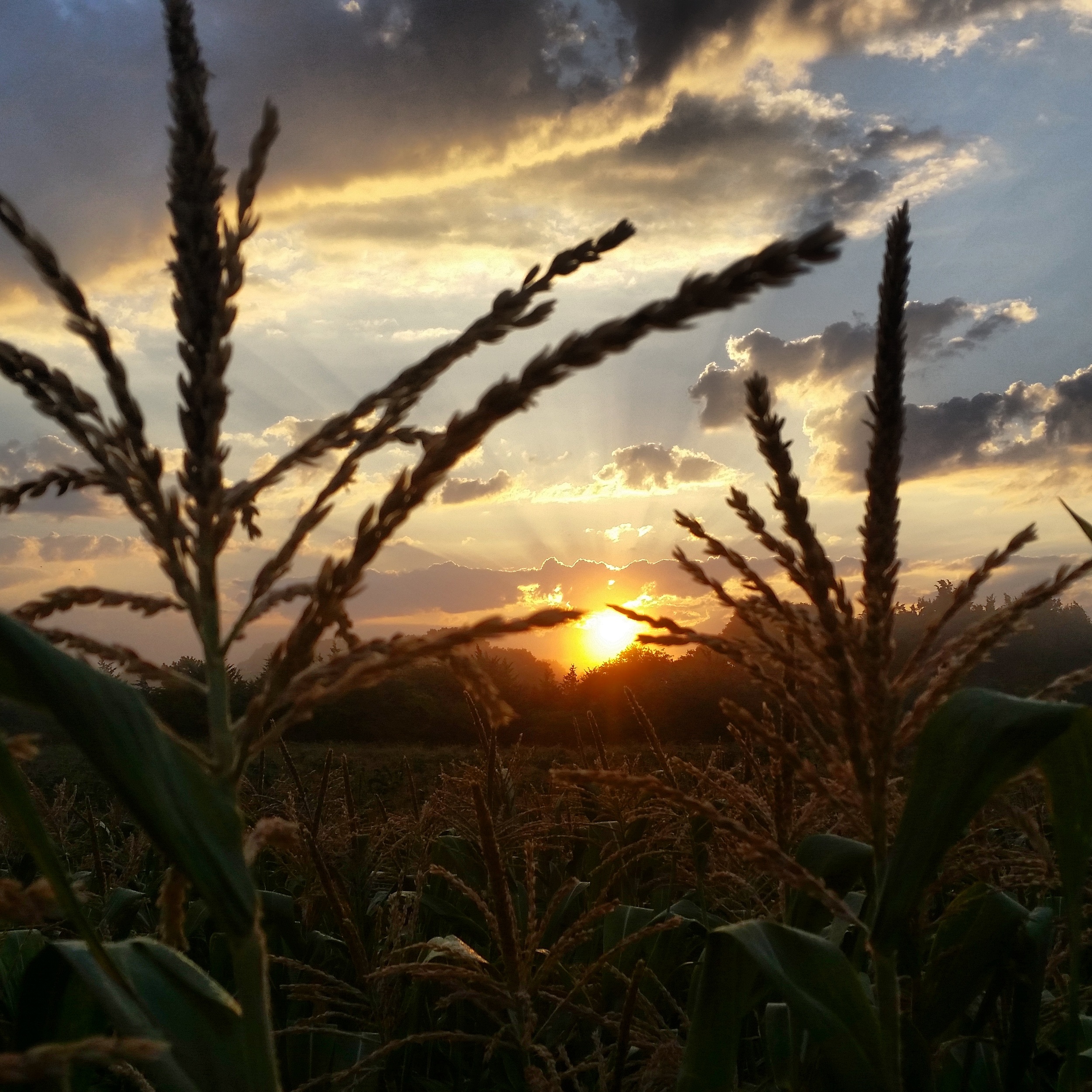A stunning photograph captures a sprawling cornfield just as the sun is setting, casting a dramatic scene. The sun, positioned almost centrally in the image, is a bright white orb surrounded by a buttery yellow halo that emits radiant rays across the partly cloudy sky. The sky itself is a dynamic mix of large gray clouds and patches of blue, with hints of orangish tones suggesting the sun's descent. In the background, a row of silhouetted trees marks the horizon, partially obscuring and emphasizing the glowing sun. The foreground showcases the tops of tall cornstalks, with their tassels prominently silhouetted against the sky, creating a textured, almost silhouette-like effect. The photo, skillfully composed, balances the dark browns and greens of the corn plants with the luminous sky, emphasizing the vastness of the field that stretches back to the tree line where the sun is nestled.